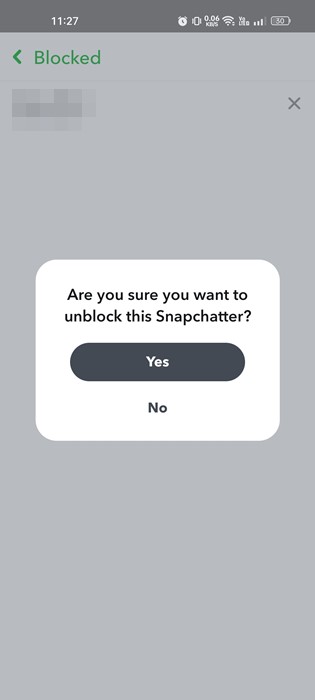The image displays a smartphone screen with various elements. In the upper left-hand corner, the time is shown as 11:27. The upper right-hand corner features multiple icons: an alarm icon, a possible vibration icon, an unknown number, a cell signal icon, a WiFi icon, and a battery icon indicating a 30% charge. Below this, there is a line with a green arrow pointing left and the word "Blocked" next to it. The subsequent line is obscured, similar to how TV censors might obscure offensive content, and marked with an 'X'.

Dominating the main portion of the image, which is set against a gray background framed by a white border, a prompt reads, "Are you sure you want to unblock this Snapchatter?" with options for "Yes" or "No". The entire image is primarily in shades of gray, black, and white, with the only color elements being the green arrow and the word "Blocked". The image captures a straightforward, monochromatic interface related to Snapchat’s blocking and unblocking feature.